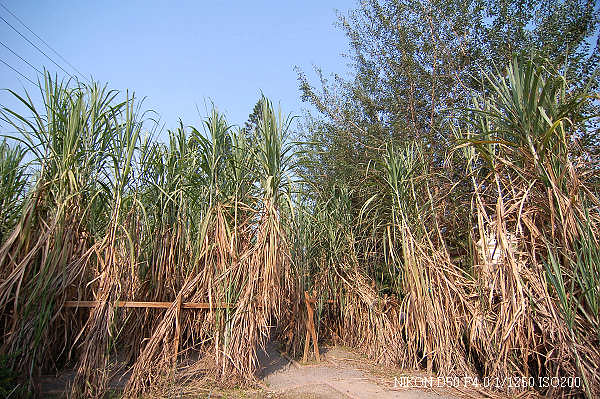This photograph captures a dense cluster of tall, cane-like plants that resemble corn stalks with a mix of dead straw-like brown leaves on the bottom and vibrant green leaves on top, almost evoking the appearance of palm fronds but shorter. The sandy brown ground is partially visible, accentuating the distinctive foliage. A narrow path weaves into the dense growth, adding a touch of mystery. To the extreme right, a larger tree extends upwards, partially obscuring the right side of the clear, blue, cloudless sky. On the far left, black telephone lines cross over the tops of the plants, while a low wooden fence with a single slat peeks through the foliage, hinting at the landscape’s boundaries.